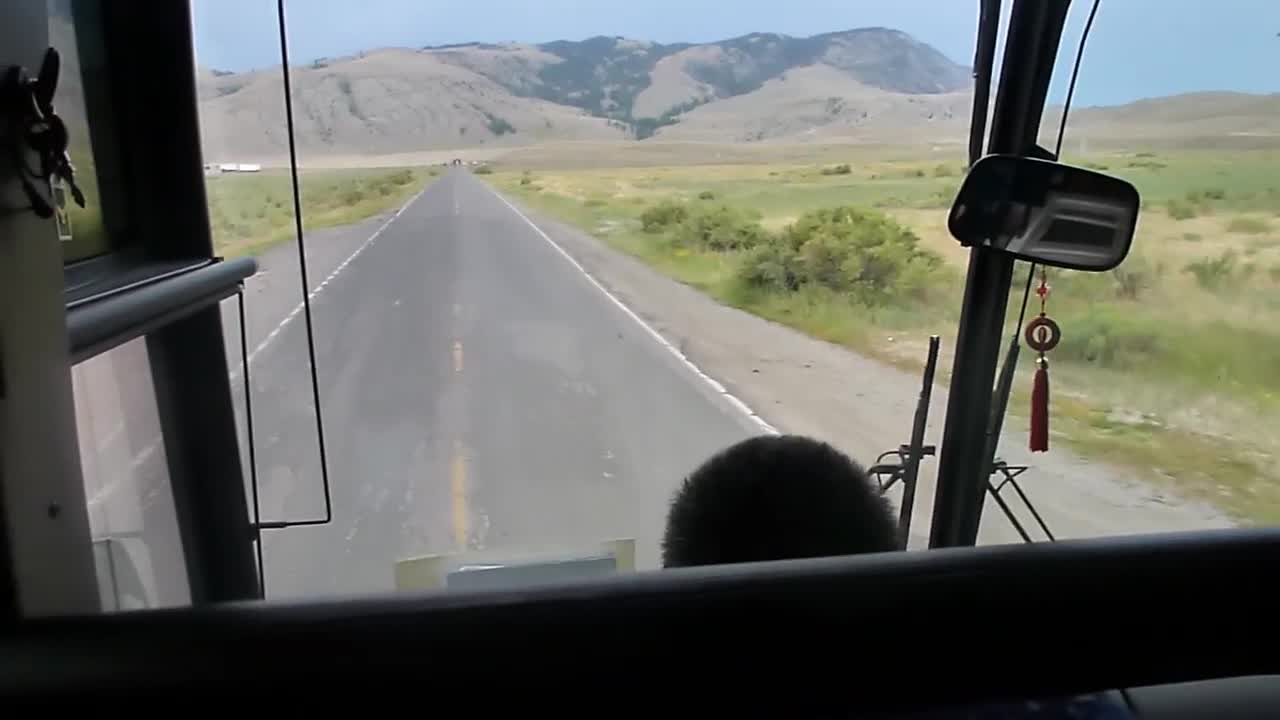The image appears to be a computer-generated scene viewed from inside a vehicle, possibly a truck. The perspective suggests that the viewer is looking slightly downward and to the left, indicating a position above the driver's seat. Visible on the left are the black frames of several windows, reinforcing the impression of a truck cabin. The driver is depicted with very short black hair and slight stubble on his scalp. Hanging from the rearview mirror is a red tassel attached to a medallion.

Outside the windshield, a two-lane gray highway stretches ahead with yellow dotted lines separating the lanes and solid white lines marking the edges. Flanking the road are patches of dry grass and bushes. In the distance, grey mountains rise up under a blue sky. Despite the detailed rendering, the overall scene outside the window has an artificial quality, suggesting it may be computer-generated rather than a real photograph.